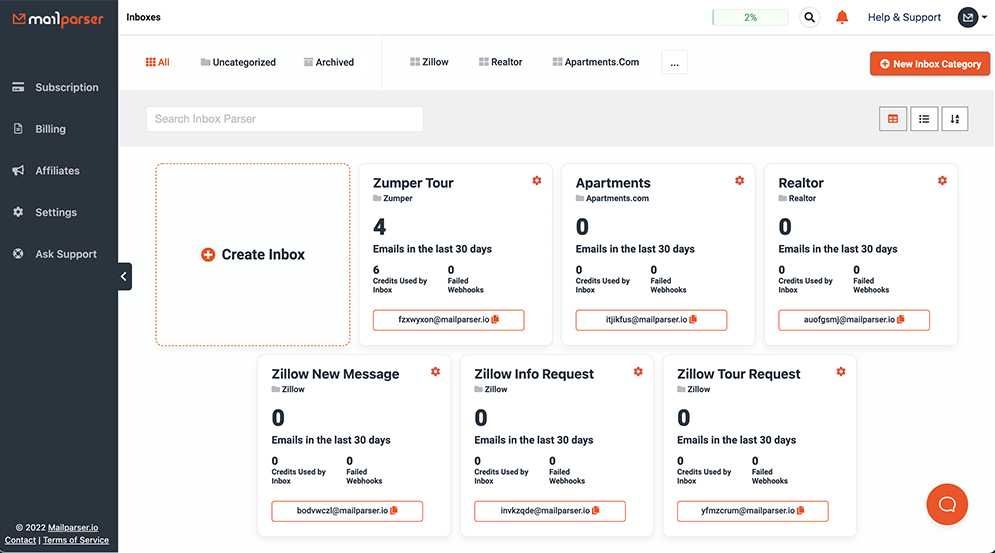The image depicts a screenshot of an email management program called MailParser. In the upper left-hand corner, the program's name is displayed, with "Mail" in white and "Parser" in orange, accompanied by a small orange envelope icon. The interface includes various categories to organize emails: Inbox, Uncategorized, Archived, Zillow, Realtor, Apartments.com, and Zumper, indicating a comprehensive management system.

The screenshot shows that 2% of the mailbox capacity is filled. Key features include a search bar, notification icon, help and support options, and the ability to create a new inbox category through a white box with an orange dotted line and a small orange plus icon labeled "Create Inbox."

The image also details email statistics for the last 30 days across different categories: "Apartments" emails, "Realtor" emails from the last day, "Zillow - New Messages," "Zillow - Info Request," and "Zillow - Tour Request." Additionally, it shows that six credits have been used and there are failed webhooks notifications.

On the bottom right, an orange chat bubble allows users to access chat support. The dark blue sidebar on the left offers navigation options for Subscription, Billing, Affiliates, Settings, and support inquiries. At the bottom right corner, legal links for Contact and Terms of Service are visible, along with the year 2022 and MailParser.io branding, suggesting that this is a subscription-based email service.